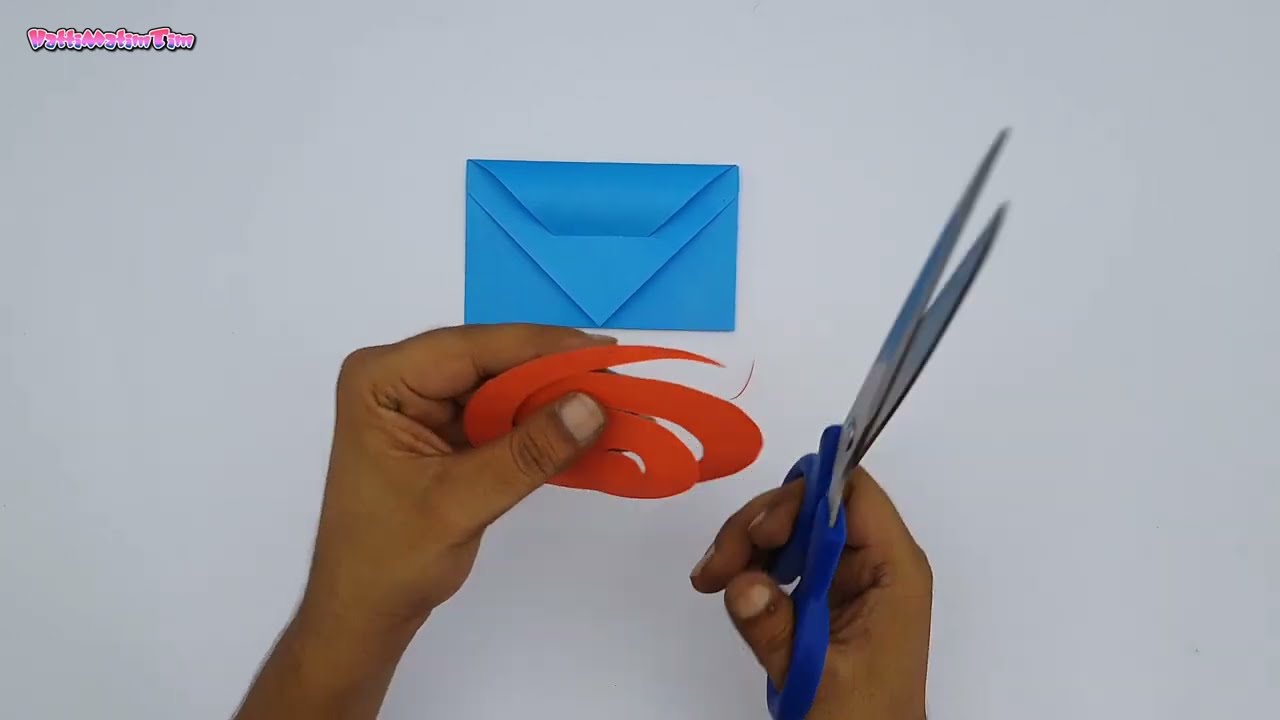In this high-definition photograph, two brown hands are prominently featured against an off-white background, which may be computer-generated or possibly a table. The right hand grasps a pair of scissors with a blue handle, poised as if mid-cut. The left hand holds an orange spiral-shaped piece of paper, clearly cut by the scissors. Centered just above the hands is a blue envelope, its top flap neatly tucked into a secondary flap. In the upper left corner of the image, there is text written in puffy pink letters outlined in black, which reads "Hattie Matt Tim Tim," though the text might appear slightly differently to some viewers. The image's details, including the precise positions and colors of the objects, contribute to a striking and focused composition.